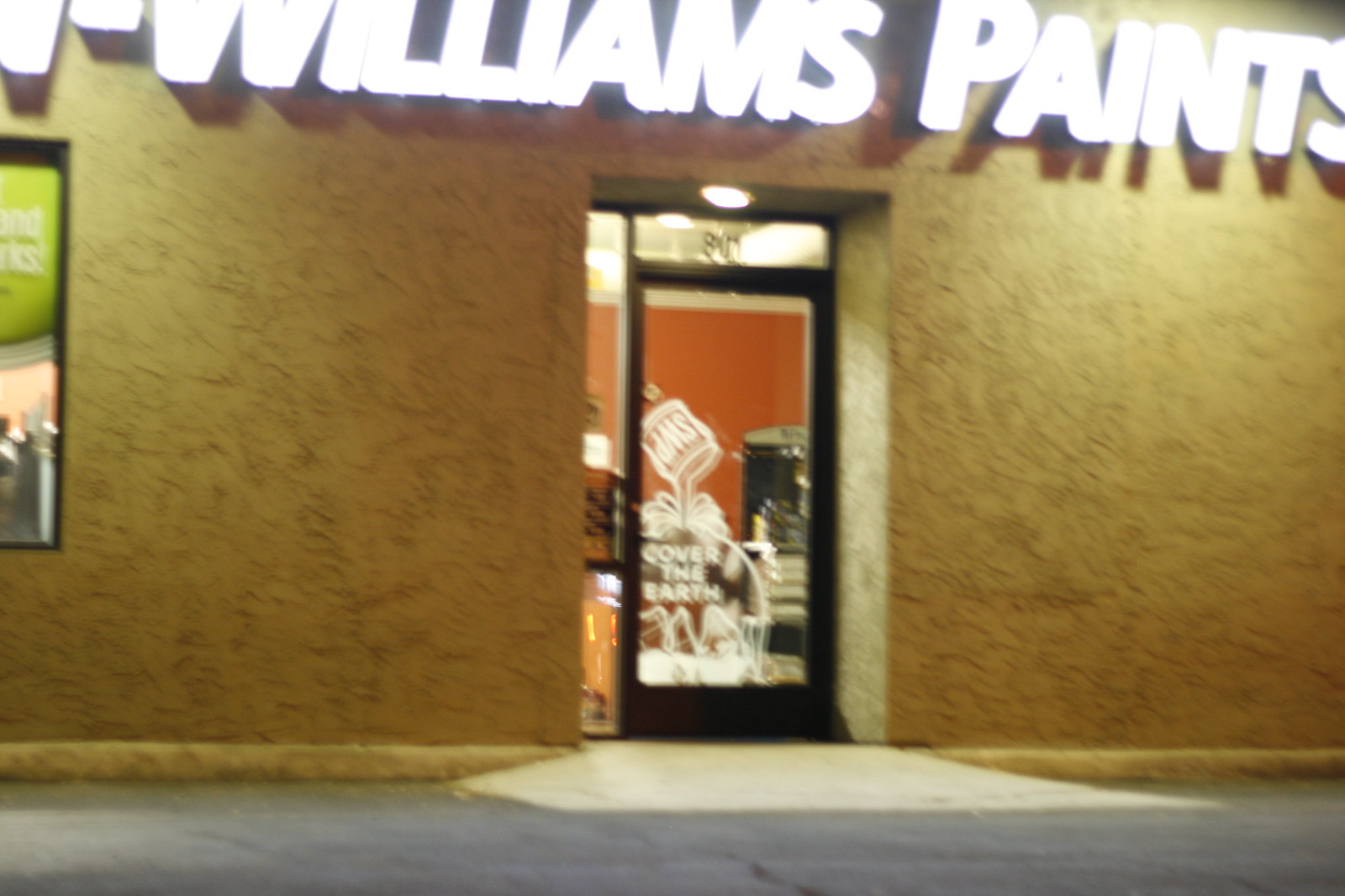This photograph, taken in landscape orientation, captures the entrance to a paint store. The image is slightly blurry, yet several details are still discernible. The bottom fifth of the photograph showcases a grey concrete surface that likely forms the sidewalk or entrance path. Above this, the building facade features a heavily textured, yellow stone concrete surface that adds a distinctive character to the storefront.

At the top of the image, a partially visible, brightly illuminated sign displays the store's name in capital letters: "WILLIAMS PAINTS." The fluorescent white letters cast subtle shadows on the building facade, further emphasizing their presence.

Central to the photograph is a glass doorway with a black frame, likely the main entrance to the store. The door bears a blurry number at the top, presumably the store’s street address. Inside, just beyond the door, there stands a promotional display featuring a paint can with a white outline. The can appears to be pouring paint, accompanied by the phrase "Cover the Earth." This eye-catching display highlights the store's core product and slogan.